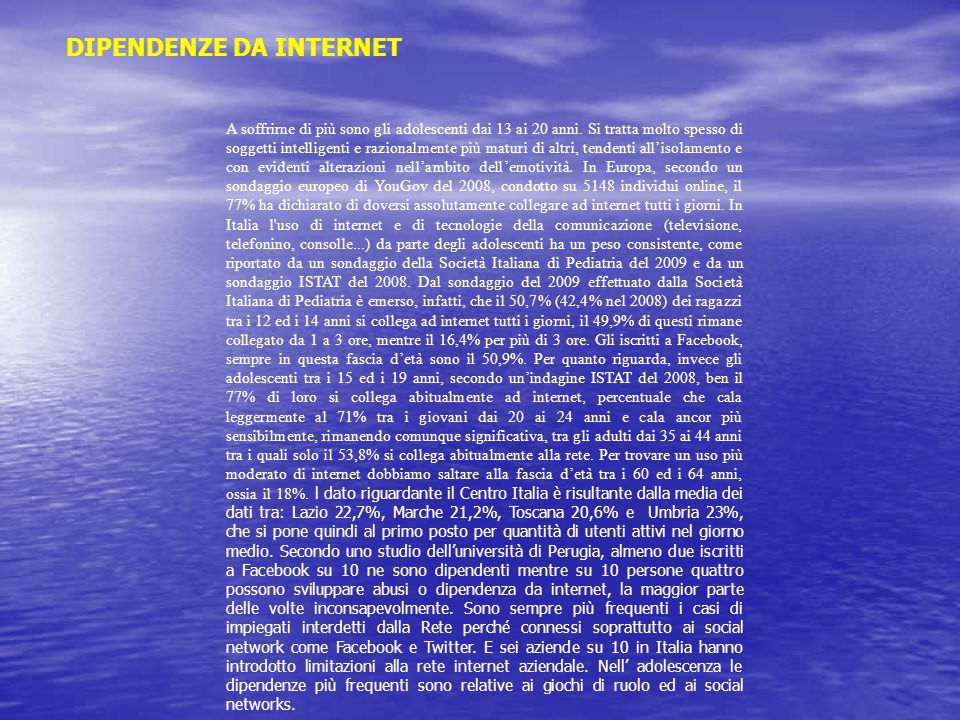The image is designed to resemble an informational slide, with a pictured background featuring an expansive blue ocean leading up to a clear sky dotted with white clouds. On the top left, the bold, yellow, all-uppercase text reads "DEPENDENZA DA INTERNET." Below this title, a lengthy block of white text spans the center of the image. This text, presumably in Italian, discusses the impact of Internet dependence on adolescents aged 13 to 20, mentioning statistics and findings from European and Italian studies conducted in 2008 and 2009. The text includes various figures and percentages, particularly emphasizing a 77% statistic, and becomes larger in font size toward the bottom. The overall layout and style suggest that this is educational content likely sourced from or intended for online dissemination. The background's serene ocean and sky contrast with the serious tone of the message about Internet dependency.